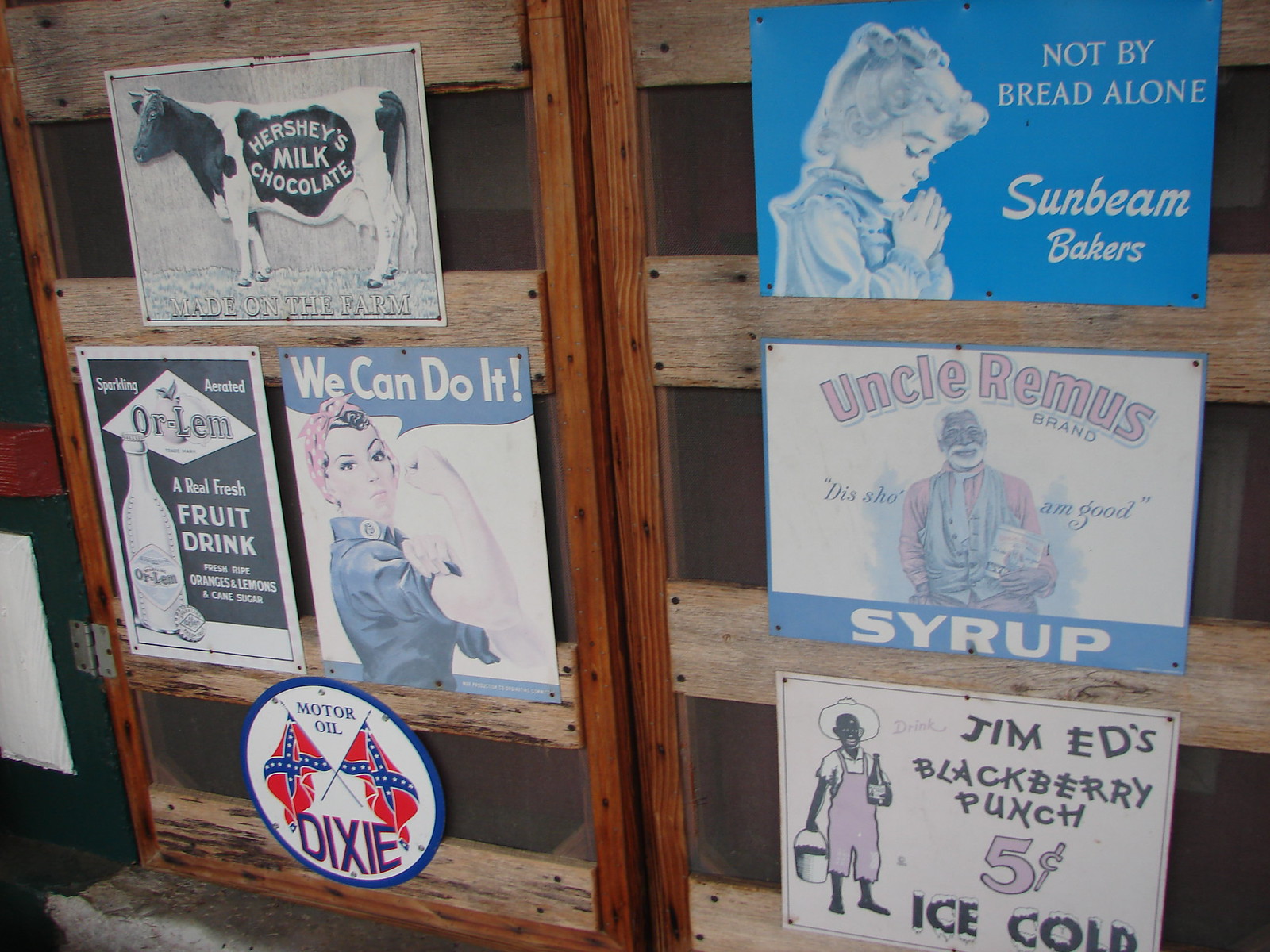This image captures a rustic wooden wall, possibly formed from window screen doors or wooden planks, adorned with a variety of vintage metal signs and plaques, their weathered surfaces displaying a glimpse into early 20th-century American advertising. Each door has dark brown frames with light brown horizontal slats, adding to the weathered ambiance.

Prominently featured is a sign for "Hershey's Milk Chocolate" depicted on a black-and-white image of a cow. The classic World War II poster of Rosie the Riveter, with the slogan "We Can Do It," showcases a strong woman rolling up her sleeves. Nearby, an old advertisement for a fruit drink boasts "Fresh ripe oranges and lemons and cane sugar, a sparkling aerated drink."

Amid these are several racially insensitive Jim Crow era signs: one for "Jim Edd's Blackberry Punch" priced at five cents with an African American character holding a drink and a bucket, and another promoting "Uncle Remus Syrup" with the slogan "This sure am good syrup." There is also a controversial "Dixie Motor Oil" sign featuring two Confederate flags. Above all, another sign shows a little girl praying with the phrase "Not by bread alone" and the logo for Sunbeam Bakers. 

These diverse, aged advertisements collectively construct a vivid, albeit troubling, portrayal of American history and pop culture.